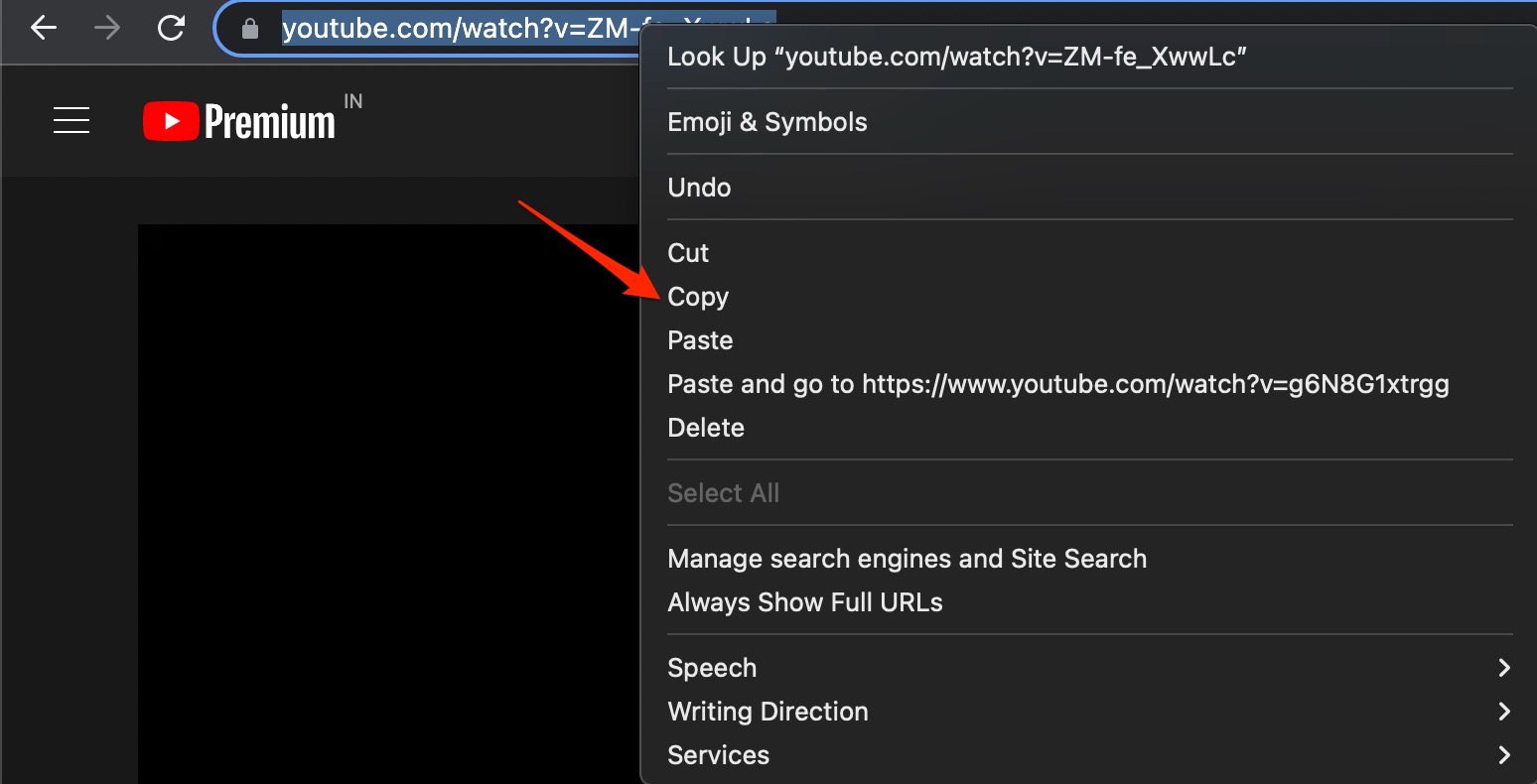This image is a screenshot from YouTube Premium. The background color is a very dark gray, almost black. On the left side, the YouTube Premium logo is displayed. The logo consists of the familiar red YouTube icon, which is a red square with rounded corners and a white play button (a triangle pointing to the right), followed by the word "Premium" written in a white font. 

Just above the "Premium" text, in a slightly lighter gray, are the letters "IN". To the left of the YouTube Premium logo, there are three horizontal white lines indicating a drop-down menu.

At the very top of the image, the website URL for a specific YouTube video is visible. The URL is shown in white font against a blue background and reads "youtube.com/watch?" followed by a unique series of letters, underscores, and numbers specific to the video.

On the right side of the image, a drop-down menu is displayed. This menu is written entirely in white font and includes several options: "Look up 'youtube.com/watch?...'", "Emojis & Symbols", "Undo", "Cut", "Copy" (highlighted with a red arrow pointing to it), "Paste", "Paste and Go to 'youtube.com/watch?...'" (where the URL differs slightly), "Delete", "Select All" (in a lighter gray font), "Manage Search Engines", "Always Show Full URLs", "Speech", "Writing direction", and "Services".